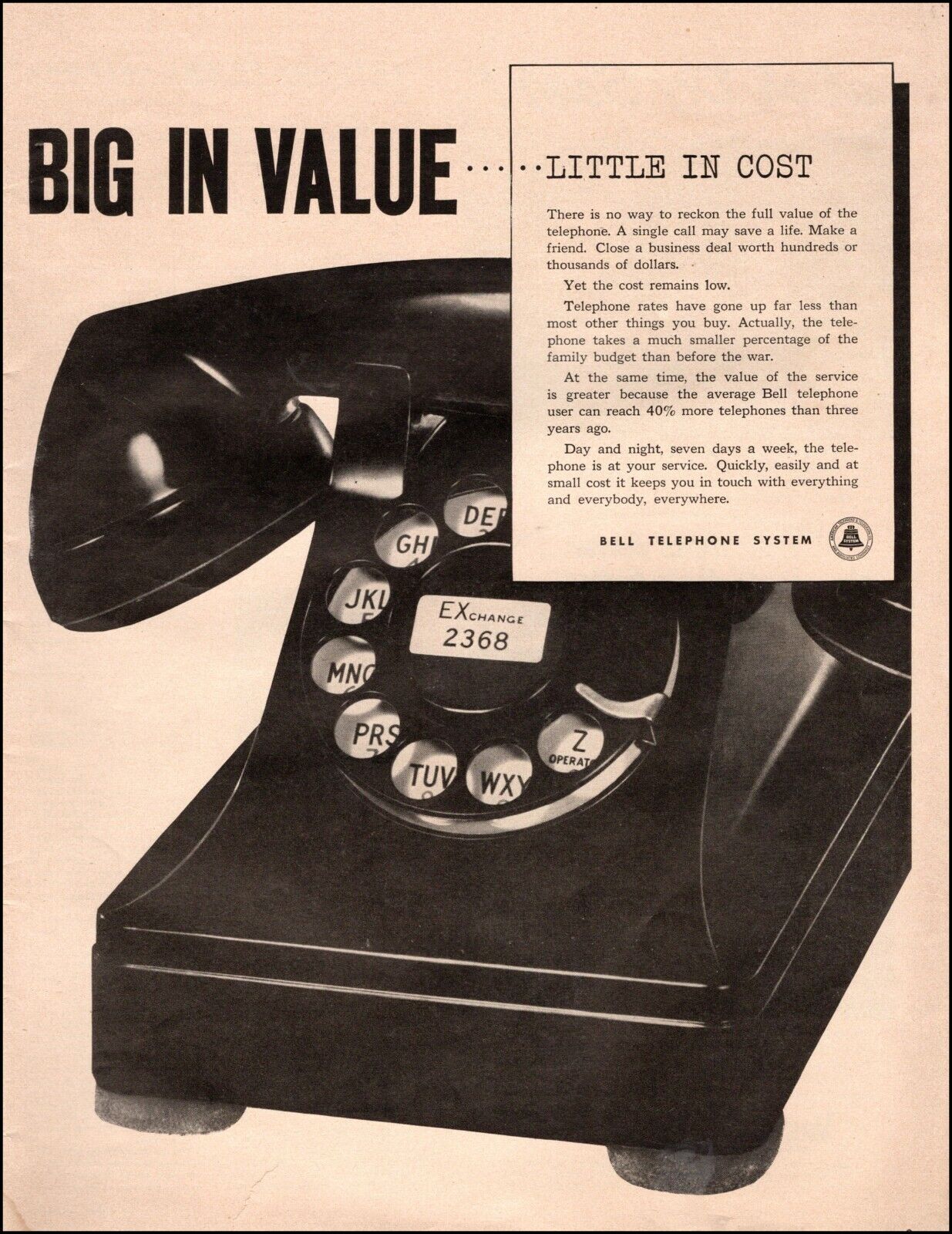The image is a vintage black and white advertisement for the Bell Telephone System, likely from the era when the telephone was a relatively new invention. Dominating the advertisement is an old-school black rotary telephone, with its handset resting atop the main body. The rotary dial prominently features a white sticker inscribed with "E-X change 2368" at its center.

At the top of the advertisement, bold black text declares "Big in value," followed by several ellipses and the phrase "little in cost" in less prominent typeface. The text highlights the significant benefits of using a telephone, emphasizing its value in daily life, such as saving lives, making friends, and closing business deals, all at a low cost. The ad also notes that telephone rates have remained relatively stable compared to other costs, and highlights that an average Bell telephone user can now reach 40% more telephones than before the war.

In the bottom right corner of the advertisement is the Bell Telephone System logo, reinforcing the brand's reliability and extensive service reach. The background of the ad is pink, providing a soft contrast to the detailed black and white imagery of the telephone and text. The phone is supported underneath by small grey structures, which may be part of the display setup. Overall, the ad aims to underscore the indispensability and affordability of the telephone service provided by Bell.